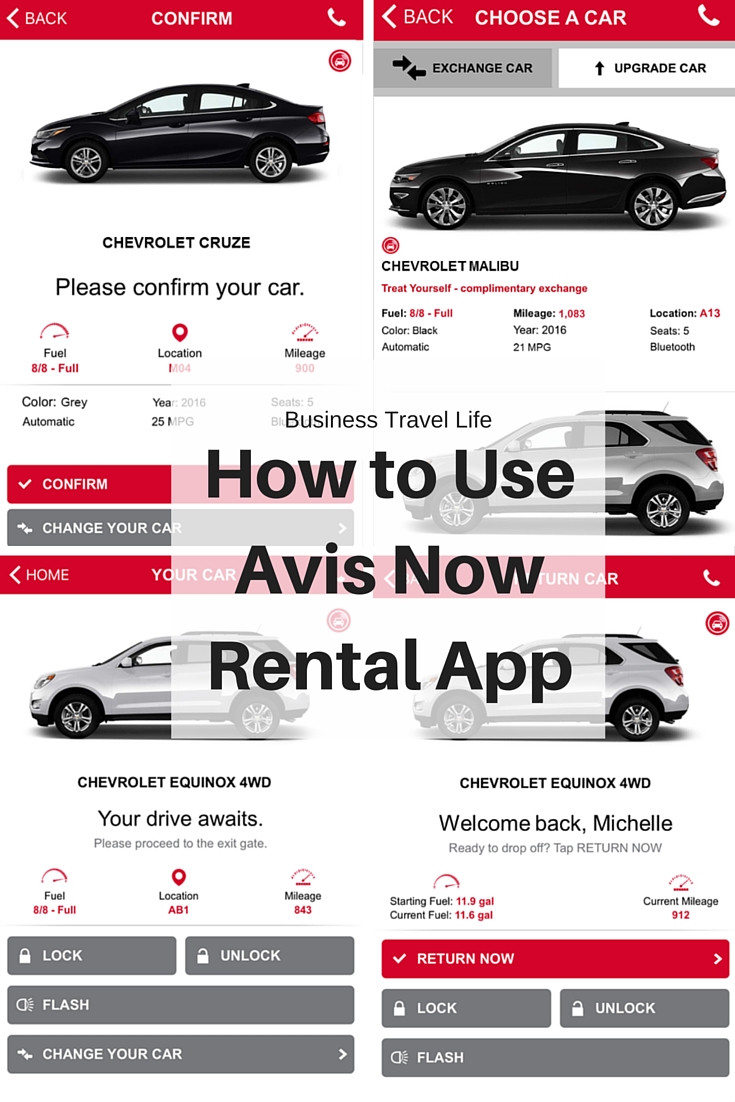**Title: Business Travel Life: How to Use the Avis Now Rental App**

The image is divided into two sections, with a central title reading in bold black text: “Business Travel Life: How to Use Avis Now Rental App,” indicating an instructional guide for the Avis rental app.

**Left Side: Picking Up Your Car**
On the left side, at the top, there is a red header with white text asking the user to "Please confirm your order." Below this header, a black Chevrolet Cruze is displayed, facing towards the left. The background for this part is white and contains detailed car information:
- Fuel: 8.8 (full)
- Color: Gray
- Transmission: Automatic
- Year: 2016
- Mileage: 900 miles
- Location: M04
- Fuel efficiency: 25 miles per gallon
- Seats: 5

There are buttons below the information for actions:
- **Confirm** (red button)
- **Change Your Car** (gray button)

Underneath, additional options are provided:
- **Home**
- **Your Car**: Chevrolet Equinox, four-wheel drive, prompting "Your driver awaits. Please proceed to exit gate." Action buttons include:
  - Lock
  - Unlock
  - Flash
  - Change Your Car (all in gray)

**Right Side: Returning Your Car**
On the right side, the header reads "Choose Your Car" in the same format. Featured is a Chevrolet Malibu with the tagline "Treat Yourself, Complimentary Exchange" in red text. This section details similar information:
- Mileage: 1,083 miles
- Location: 818
- Seats: 5
- Bluetooth
- Year: 2016
- Fuel efficiency: 21 miles per gallon
- Transmission: Automatic

Below, a gray car image is labeled “Return Car,” with a red button to initiate the return process:
- **Return Car** (red button)

Further below, another car graphic, similar to the one from the left side, labels "Welcome Back, Michelle, Ready to Drop Off," directing to "Tap Return Now" with a red “Return Now” button. Additional actions are displayed in gray:
- Lock
- Unlock
- Flash

The left side predominantly handles the car pickup process, while the right side focuses on the car return process.